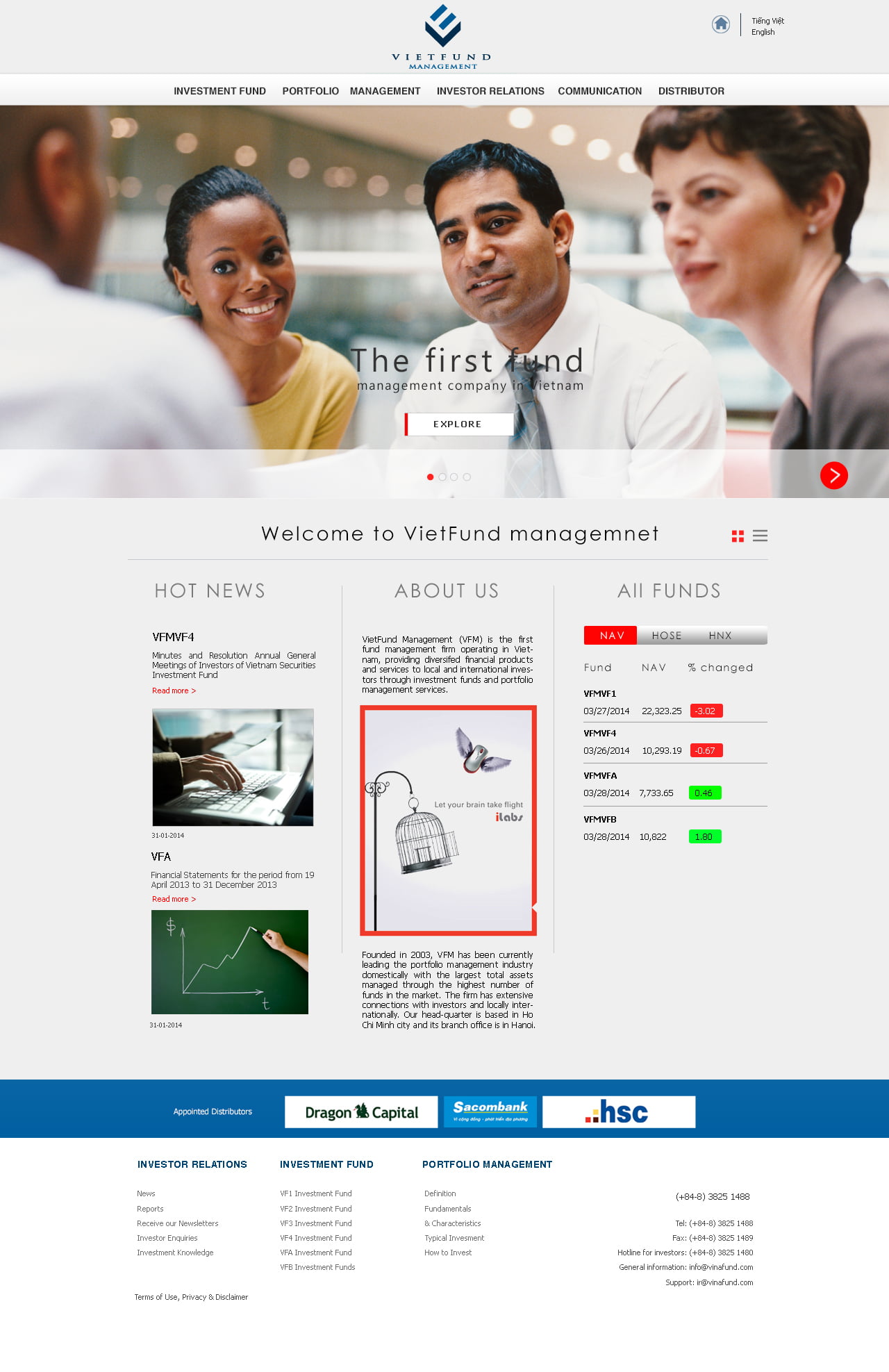The image has a light blue background with various elements arranged across it. At the top, there's a light blue box containing a sideways "E" symbol and the word "Visit." Next to this, inside a circle, there is a star enclosed by a line, accompanied by other blue text. Several headings follow below this area. 

Dominating the center of the image is a large picture of four people—two men and two women—with the words "The First Fund" printed above them. Below this image, there is a search box. Underneath the search box, a thin line features a small red dot, leading to a larger red circle containing a right arrow and the text "Welcome to Veal Fund Management." Surrounding the circle are four small red dots and three lines.

To the left of the large picture, there are sections titled "Hot News," "About Us," and "All Funds." The "Hot News" section features two pictures with accompanying articles, each overlaid with red text. The "About Us" section is centered and bordered in red, showcasing an image of what seems to be a bird or a flying insect, likely a bird in a cage.

On the right side of the image, within the "All Funds" section, there are red and white text areas, along with red and green boxes. At the bottom, a long blue box labeled "Oregon Capital" is displayed beside a white box, followed by another blue box and a white box labeled "HSC." Beneath these, there is a white area listing numerous names.